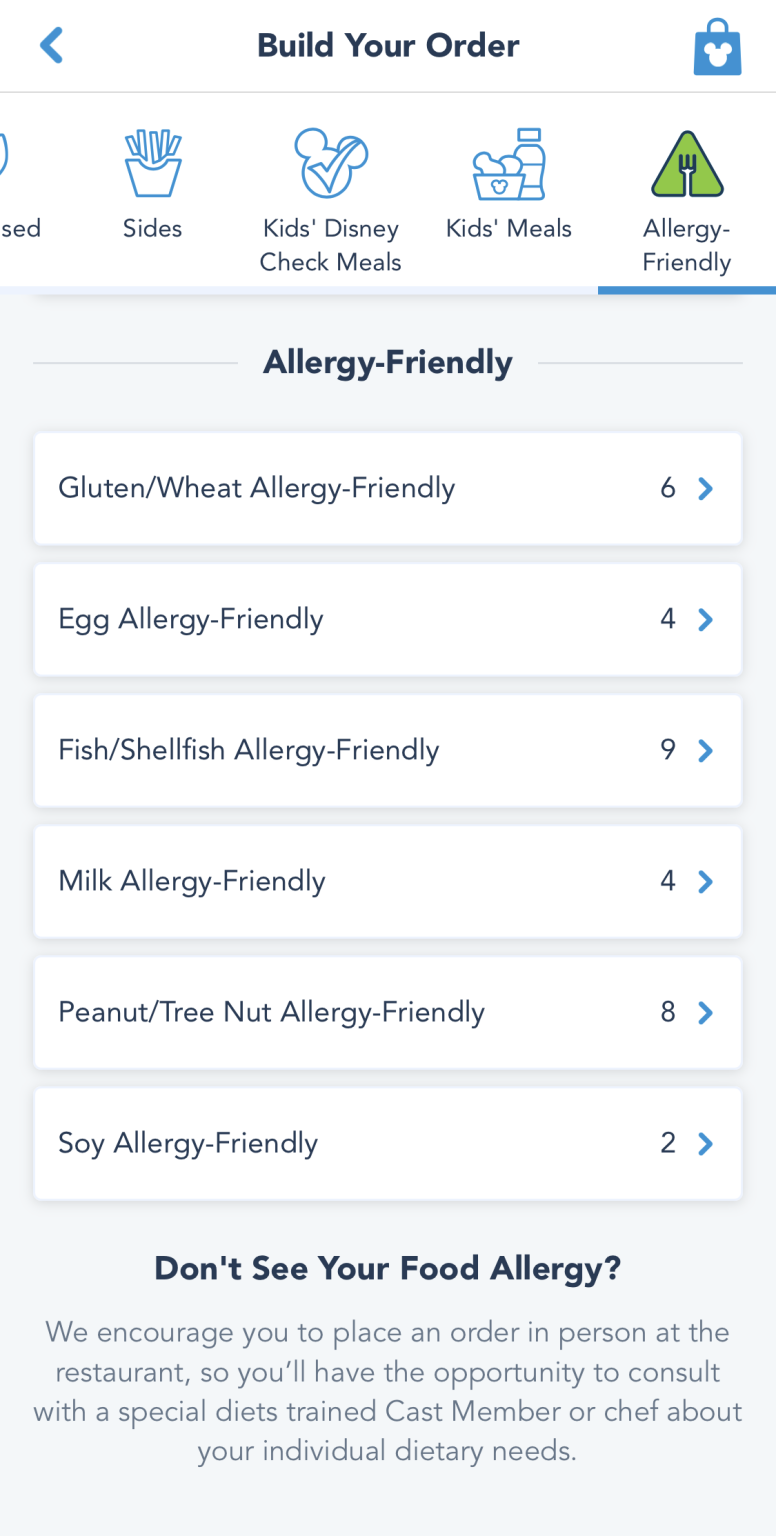The image depicts a screenshot from a food ordering application. At the top of the screen, there is a header that reads "Build Your Order" in black text. On the top right corner, there's an icon of a blue gift bag adorned with a white Mickey Mouse insignia. On the top left, there's a back button to navigate to the previous screen.

Below the header, there are several category options for building a meal:
- "Side" on the left side is represented by a blue illustration of fries.
- "Kids" features a blue icon of Mickey Mouse with a checkmark.
- "Disney Czech Meals" appears next with an associated Mickey Mouse icon.
- "Kids Meal" on the top right shows icons of small bottles and food items.
- "Allergy Friendly" is highlighted with a blue underline and features a green shaded triangle icon with a fork in the center.

Under the "Allergy Friendly" section, there are six options, each detailing different allergen-friendly meals:
1. "Gluten or Wheat Allergy Friendly" indicating three available choices.
2. "Egg Allergy Friendly" with four available choices.
3. "Fish or Shellfish Allergy Friendly" offering nine options.
4. "Milk Allergy Friendly" presenting four choices.
5. "Peanuts and Tree Nut Allergy Friendly" with eight options.
6. "Soy Allergy Friendly" showing two available choices.

At the bottom of the screen, there's a message that reads: "Don't see your food allergy? We encourage you to place an order in person at the restaurant so you will have the opportunity to consult with a special diet-trained cast member or chef about your individual dietary needs."